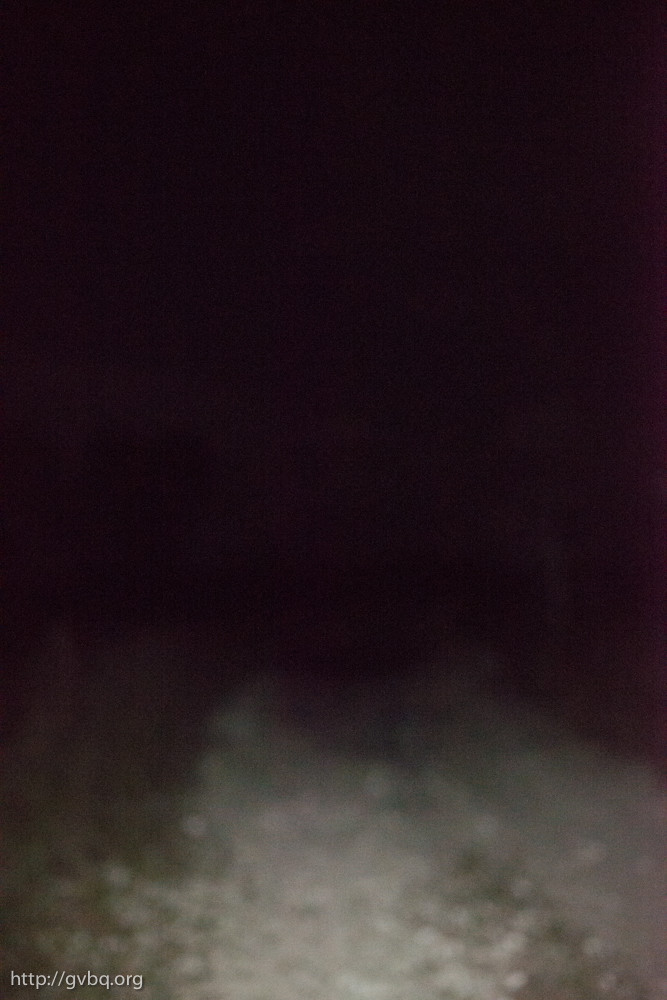This image resembles a scene from the Blair Witch Project due to its extremely low quality and dark, eerie atmosphere. Taken at night, it is predominantly pitch black from about a quarter of the way up to the top, with only the lower one-third faintly illuminated. The light barely reaches the foreground, creating a very blurry effect. The bottom portion appears grayish with white spots that blend together, suggesting either gravel or a snow-covered dirt road, but the extreme pixelation makes it difficult to distinguish the exact surface. In the bottom left corner, there is a text overlay displaying the URL "http://gvbq.org." The poor quality and focus contribute to the overall ambiguity of the scene.